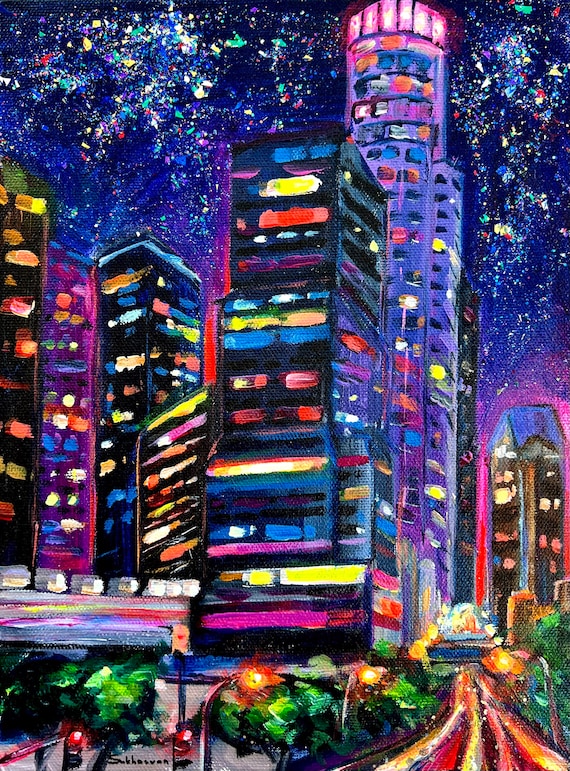A vibrant, modern painting features a night-time cityscape with a mesmerizing sky filled with swirling splotches of dark blues, purples, and bright accents of greens, reds, yellows, and whites, resembling stars or possibly fireworks. Dominating the lower two-thirds of the artwork is a sprawling city skyline of high-rise buildings and towers, each floor illuminated with an array of colors, including purples, blues, reds, and yellows. The tallest structure, with a round top, nearly reaches the top of the canvas. At the bottom right, a freeway is depicted in a time-lapse style, with streaks of light representing the flow of traffic. Trees and greenery are scattered intermittently, adding a touch of nature to the urban scene. In the bottom left corner, two bright red stoplights and tall, curved poles with glowing yellow and orange lights further enhance the city's lively atmosphere.